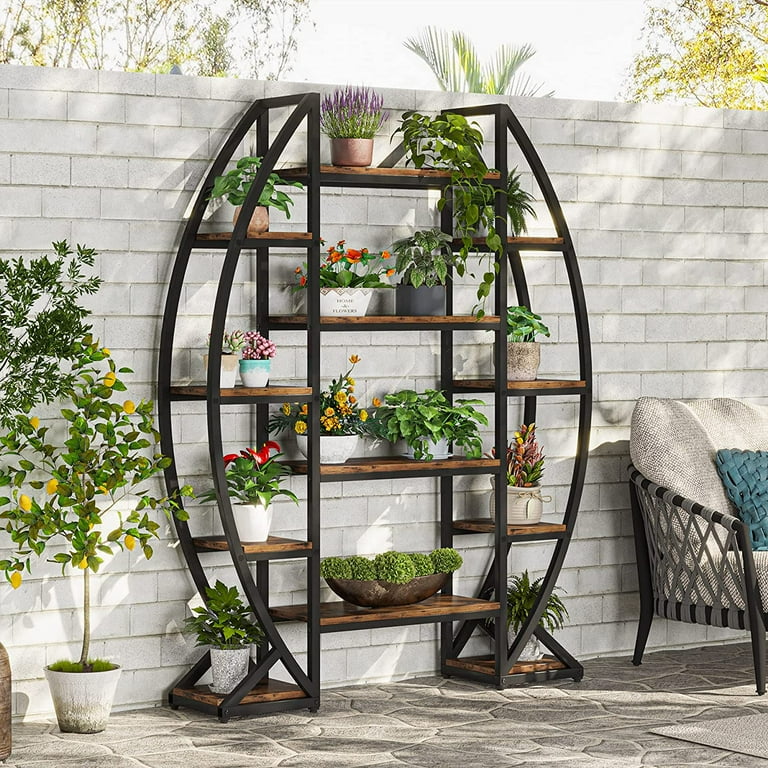The image depicts a stylish shelving unit set against a white brick wall and grayish-white brick flooring. The black metal-framed shelves, crafted from brown wood, are arranged symmetrically into three columns—each with varying shelf levels: three on the outer sides and four in the middle, totaling twelve shelves. Each shelf hosts a variety of vibrant plants in diverse vases, featuring red and yellow flowers, green foliage, and even some purple blossoms. On the left side, a small lemon tree grows in a white pot, while the right side features a white wicker bench with black metal legs, topped with a blue cushion and a gray seat cushion. This arrangement creates an aesthetic outdoor display dedicated to showcasing an array of colorful plants and flowers.